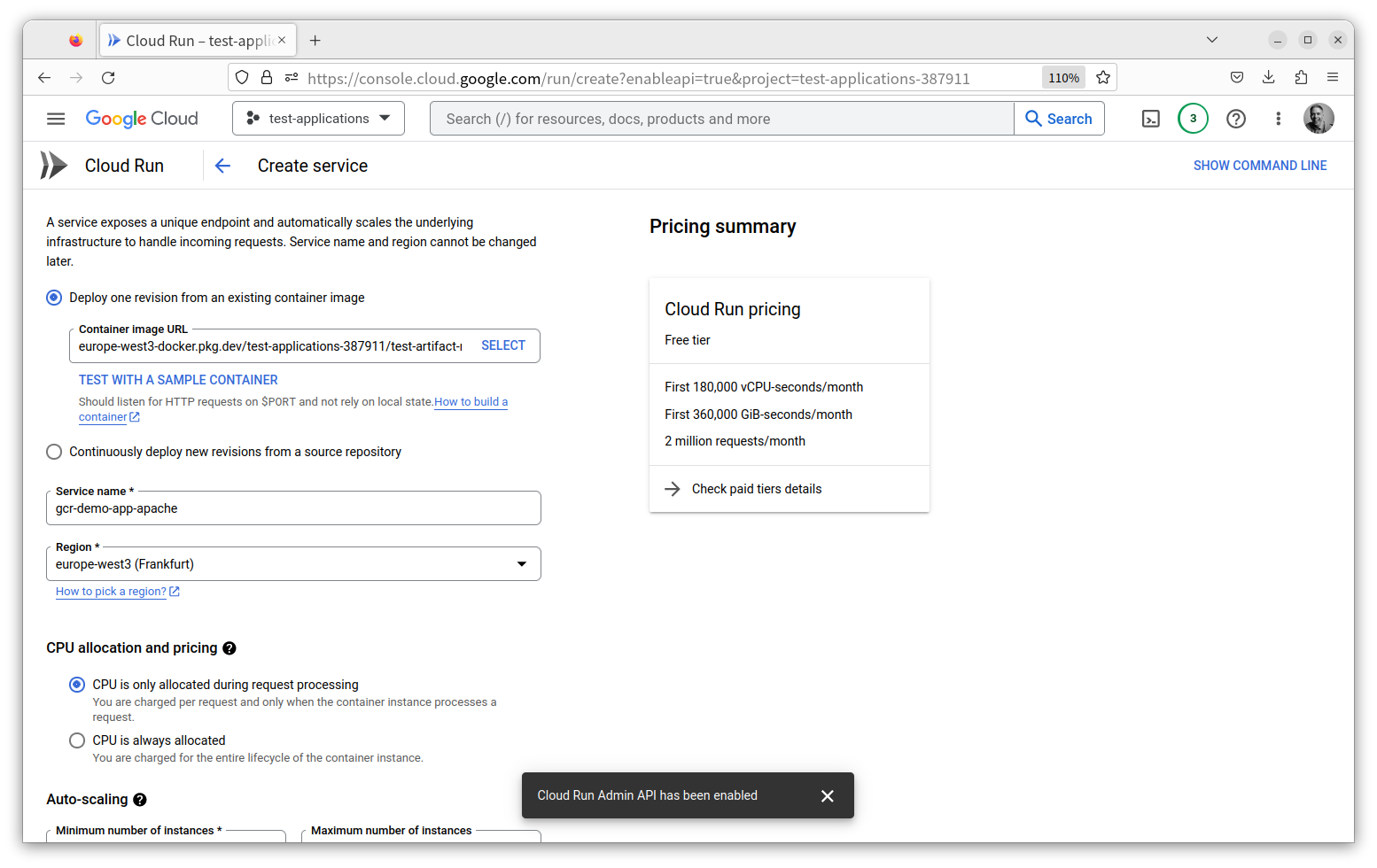The image captures a screenshot from the Google Cloud Console, specifically focusing on the Cloud Run interface where an application is being tested. At the top left of the screen, there's a prominent red record button. Adjacent to this button is a blue triangular icon, symbolizing the active tab labeled "Test App." The URL displayed in the address bar is console.cloud.google.com, indicating access to the Google Cloud Console.

The screen is zoomed in at 110%, which is evident from the level of detail visible. The interface's star icon, used to favorite the page, is empty, signifying that this Cloud Run page is not favorited. At the top of the interface, the Google Cloud logo is visible, accompanied by a search bar labeled "Search for resources, docs, products, and more," with a blue search button featuring a magnifying glass icon.

To the right of the search bar, several icons are displayed, including the user’s profile picture. Below this header, the "Cloud Run" label is prominent, with a blue arrow icon pointing towards it and a "Create Service" button next to it. The interface presents various options for deploying a cloud service. Two primary radio button options are visible: one for deploying a single revision from an existing container image (with its associated URL) and another for continuously deploying new revisions from a source repository.

Additional details include fields for server name and region selection. On the right side of the interface, information about CPU allocations and a pricing summary in bold, providing insight into the cost implications of the selected configurations, is visible.